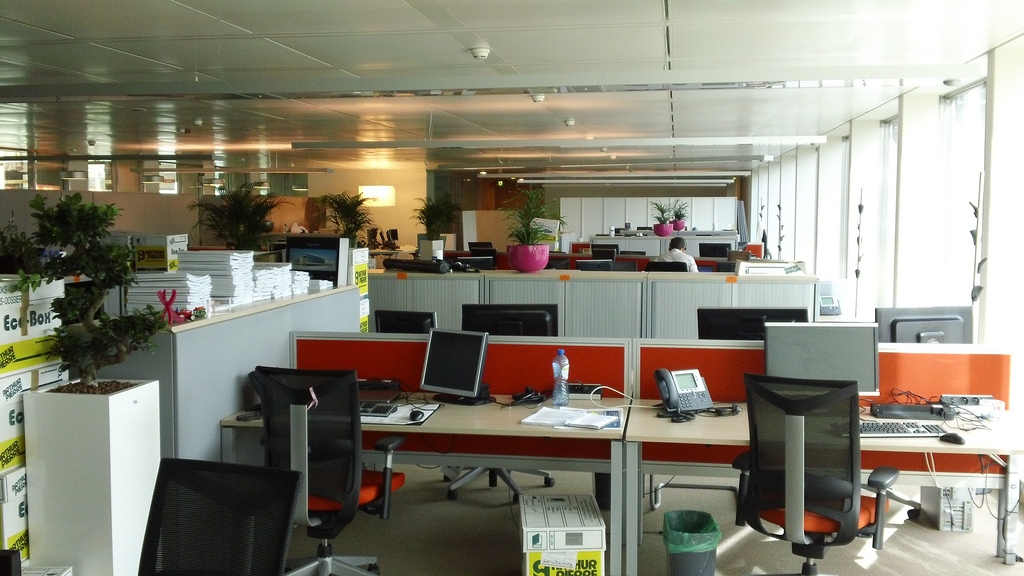The image depicts a busy office building's interior, characterized by rows of cubicles and desks arranged closely together. Dominating the right side of the scene, large windows allow daylight to flood in, providing natural illumination to the workspace, which has a ceiling composed of white tiles with built-in lights and visible fire sprinkler heads. Each cubicle contains a set of red-backed desks accompanied by black-backed chairs with red seats. Every desk is equipped with a computer monitor framed in gray, a keyboard, a mouse, and a slanted desk phone on the left side. Additionally, there's a green-insert trash can and a box with a white lid featuring yellow and green lettering on the floor. To the left, tall white pots with green plants and stacks of papers or bags are visible, contributing to a cluttered atmosphere. In the middle to upper section of the image, a single person, dressed in a long-sleeve white shirt and seated, appears to be working, gazing downward. The floor suggests carpeting with scattered wires, and the overall lighting is a mix of natural and artificial sources, maintaining a functional yet slightly congested office ambiance.